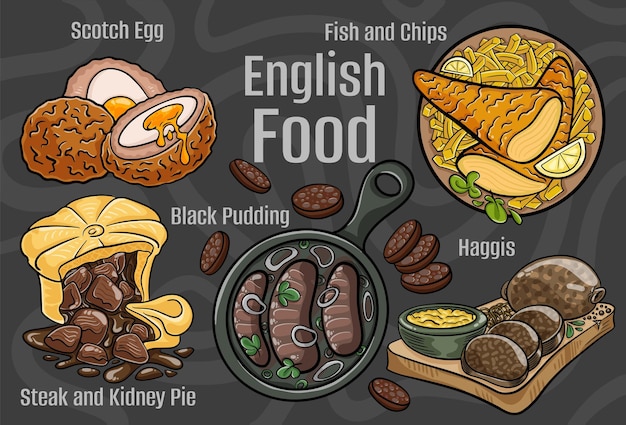This digital illustration showcases an array of quintessential English foods, all labeled with light gray text on a charcoal gray background adorned with abstract lighter gray swirls. At the center, the words "English Food" anchor the image. The upper left corner features Scotch eggs, depicted as halves with a runny yolk encased in a breaded, fried shell. Below this is a steak and kidney pie, light brown in color, sliced open to reveal dark brown pieces of steak and kidney spilling out, accompanied by a rich, dark gravy. Centrally located, black pudding is shown as dark brown sausages with lighter centers, presented in a large dark gray cast iron skillet with green garnishes. Moving to the right, the fish and chips scene includes two triangular pieces of breaded fish, beige on the inside, served with golden yellow fries, lemon wedges, and green garnishes, all arranged on a brown plate. The lower right corner depicts haggis on a brown cutting board, with slices of meat and a dip or sauce, possibly accompanied by a bowl of porridge-like substance. Each dish is meticulously detailed to highlight their unique textures and colors, providing a comprehensive visual feast of traditional English cuisine.